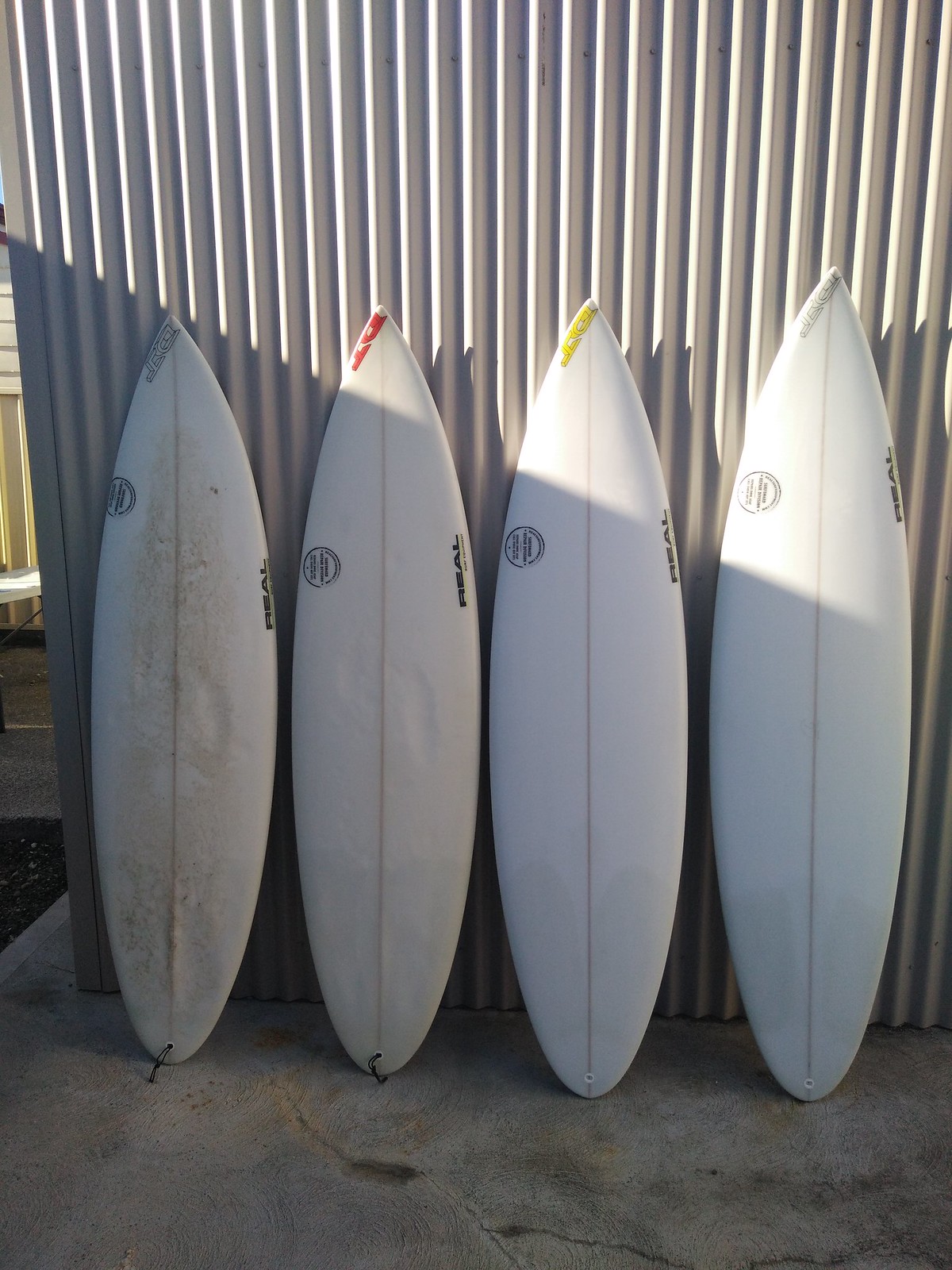The image features four white surfboards lined up and leaning against a vertically striped wall that resembles the side of a metal building, creating a backdrop with a pale, almost white, color. Each surfboard has a distinct marking at its tip: the first one has a gray marking with some text, the second tip features some red, the third shows yellow, and the fourth displays light gray. The boards also feature a vertical line down the middle and a circular marking on the upper left side. The surfboards rest on a cracked, stained concrete sidewalk, which bears signs of wear and moisture exposure. The positioning of the surfboards creates a shadowed effect at the base, with sunlight diagonally illuminating the tips of the last two boards on the right. The three on the left are the same height, while the one on the right is slightly taller. Two of the boards exhibit scuff marks and indentations where feet have been placed, indicating usage, while the other two appear to be new.